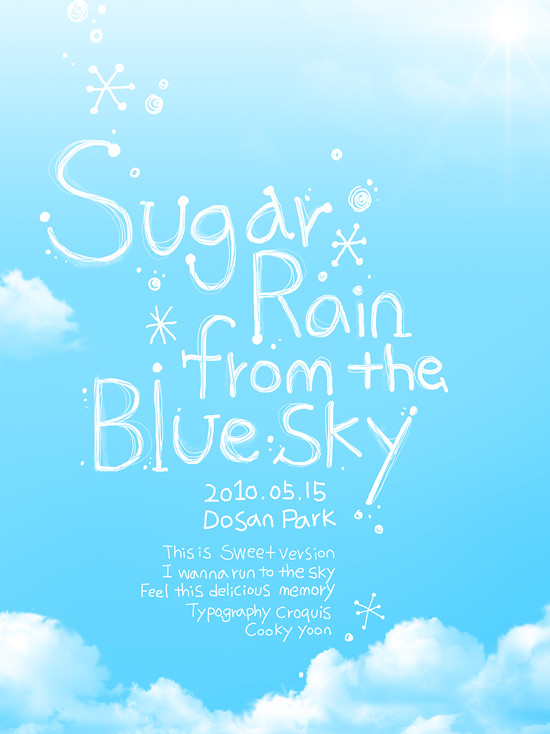The artwork, titled "Sugar Rain from the Blue Sky," showcases a light blue sky with fluffy white clouds concentrated towards the bottom left and golden light rays peeking through the top right corner. The centerpiece features large white typography stating "Sugar Rain from the Blue Sky," accented by small graphics of descending bubbles and snowflakes. Beneath this central text, in smaller white font, it reads: "2010.05.15 Dosan Park." An additional playful line adorns the piece: "This is sweet version I want to run to the sky fill this delicious memory." The font style is whimsical and cloud-like, subtly blending into the sky's background, creating a harmonious and dreamy effect. The design and additional typography credit 'Crocus' and 'CookieYou,' enriching the surreal and sweet essence of the artwork.